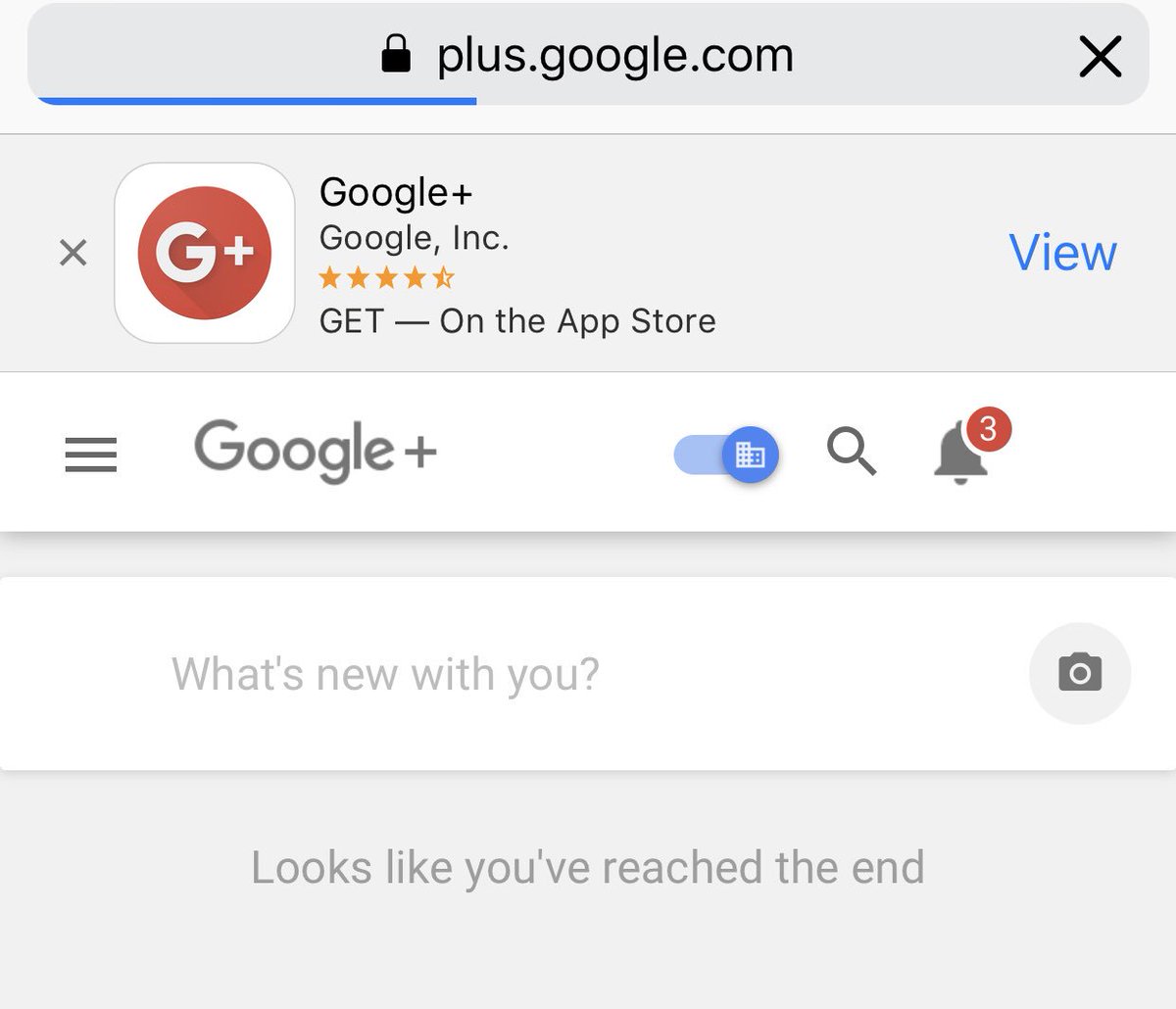This image depicts a web graphic associated with Google Plus. Dominating the top part of the image is a light gray background, centered within which is a black padlock icon accompanied by the text "plus.google.com" in black. To the right of this, a black "X" icon is visible.

Below this section, a blue horizontal line extends from the left edge up to the "L" in "Plus". Further down, the background transitions to a light gray with an X icon followed by a square with rounded corners. Inside the square is a red circle containing a capital "G" paired with a plus sign.

Surrounding this central element, black text reads "Google Plus," with the "G" capitalized. Beneath "Google Plus," the text states "Google, Inc." with a capital "G" and a period following "Inc." Next, a star rating is mentioned, followed by the bolded text "GET" (in all capital letters) after a hyphen, implying an option to "Get on the App Store." Adjacent to this, "view" appears in blue text.

Descending further, a banner with the phrase "What's new with you?" is visible, featuring a circle with a black camera icon inside. Continued below, the gray background persists, and the text reads, "Looks like you've reached the end."